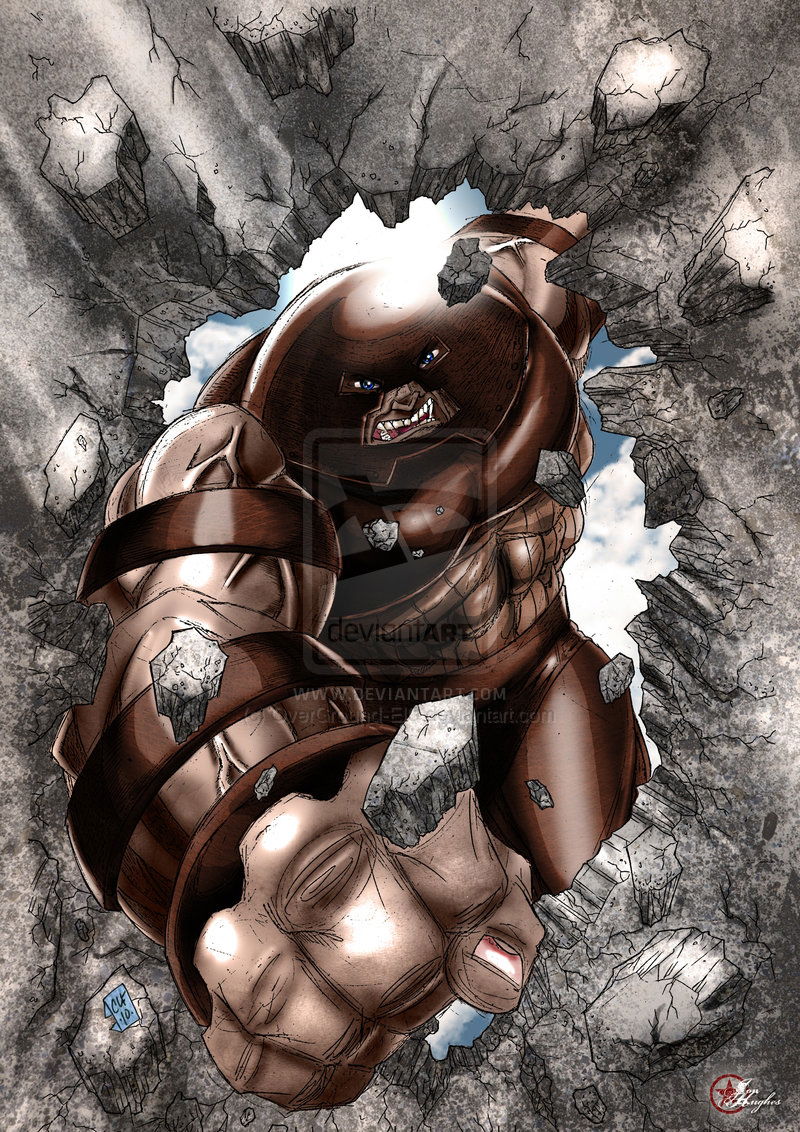This is a highly detailed, fantasy-style, poster-sized illustration of Juggernaut from the X-Men, depicted in the throes of smashing through a stone wall. The gray wall, accented with white highlights, crumbles as his balled-up fist bursts out towards the viewer, creating an explosion of flying rocks. The artwork showcases Juggernaut mid-action, his other arm poised yet to break through the barrier. Illuminated from above by sunlight, his fierce, grimacing face is framed by an egg-shaped helmet, revealing his menacing fangs and blue eyes. His broad, rounded brown head and exceptionally muscular physique—chest, arms, and legs—are prominently displayed, emphasizing his formidable strength. Behind the wall, hints of the sky and clouds add depth to the background. The piece also includes a DeviantArt watermark and artist signature at the bottom right corner, capturing the dynamic intensity and power of the moment.